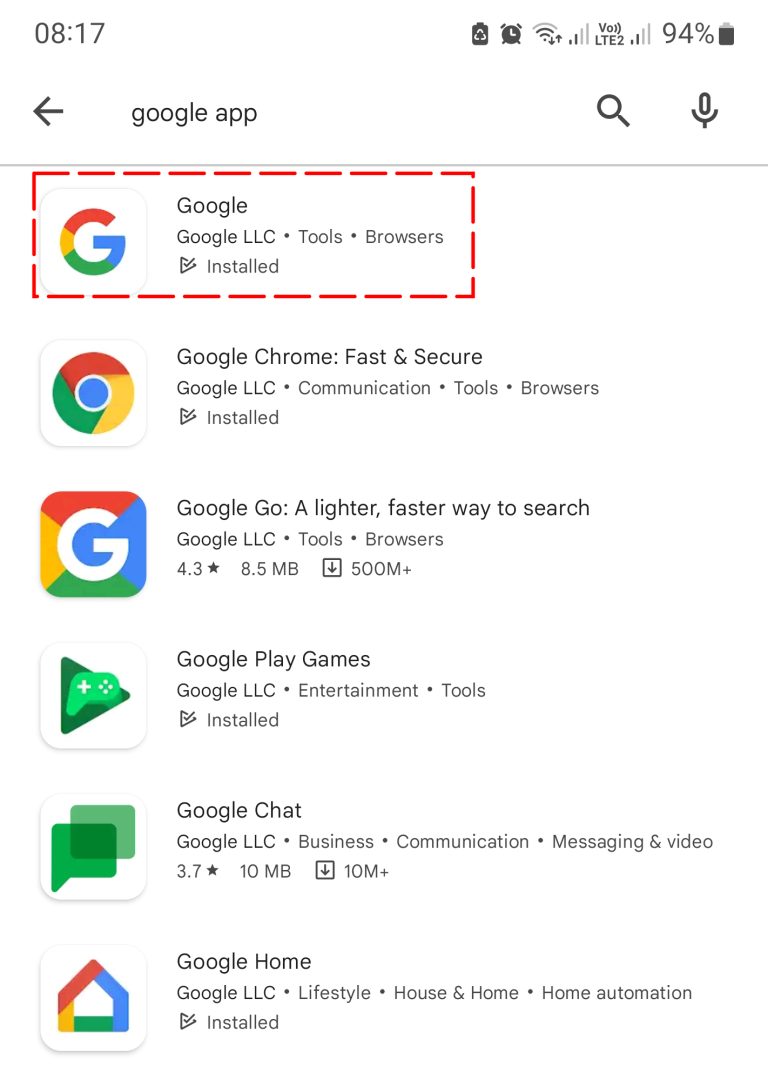The screenshot shows a mobile phone screen at 8:17 AM, as indicated at the top left corner. The top right corner displays various icons, concluding with a battery indicator showing 94% charge. Below the status bar, there's a back arrow icon followed by the words "Google app" in the search bar, accompanied by a magnifying glass and a microphone icon to its right.

Below the search bar, a list of Google-related applications is displayed. The first app is highlighted with a red dashed rectangle and labeled "Google." Next to it, "Google LLC" is listed under the categories Tools and Browsers, with a note that it is installed. The app icon, a multicolored ‘G’ on a white background, appears to the left.

The second app is "Google Chrome," with its familiar round icon featuring red, green, yellow, and blue colors. Following that is "Google Go," described as "a lighter, faster way to search," with its icon also to the left. The list continues with icons and titles for "Google Play Games," "Google Chat," and "Google Home."

The entire background of the screenshot is white. Each app title is prominent, with additional descriptive text in smaller, yet clear, black print beneath them. Each app icon is neatly placed in a square on the left side of its respective listing.